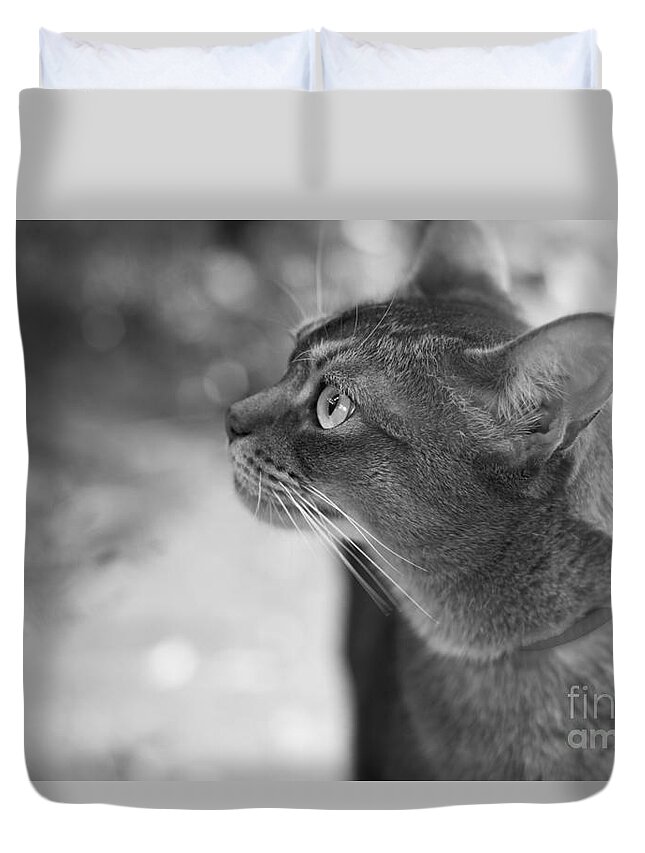This detailed aerial image focuses on a rectangular bed with a plain white background. At the top of the bed are two pillows with white pillowcases, partially covered, revealing some stains or faded grey areas. The pillows are positioned side by side. The bedspread prominently features a large, two-toned grey blanket. In the center of the blanket is a black and white print of a cat, capturing the cat’s head and chest. The cat, with a collar, is looking to the left side of the image, allowing visibility of its left profile, including white whiskers and light eyes directed upwards. The cat’s body shows minimal striping solely over the head, while the rest remains a solid light grey. The surrounding background behind the cat is blurred with light grey circular patterns, adding to the artistic effect. In the lower right-hand corner of the image, there are faint letters, "F-I-N," and below that, "A-M."